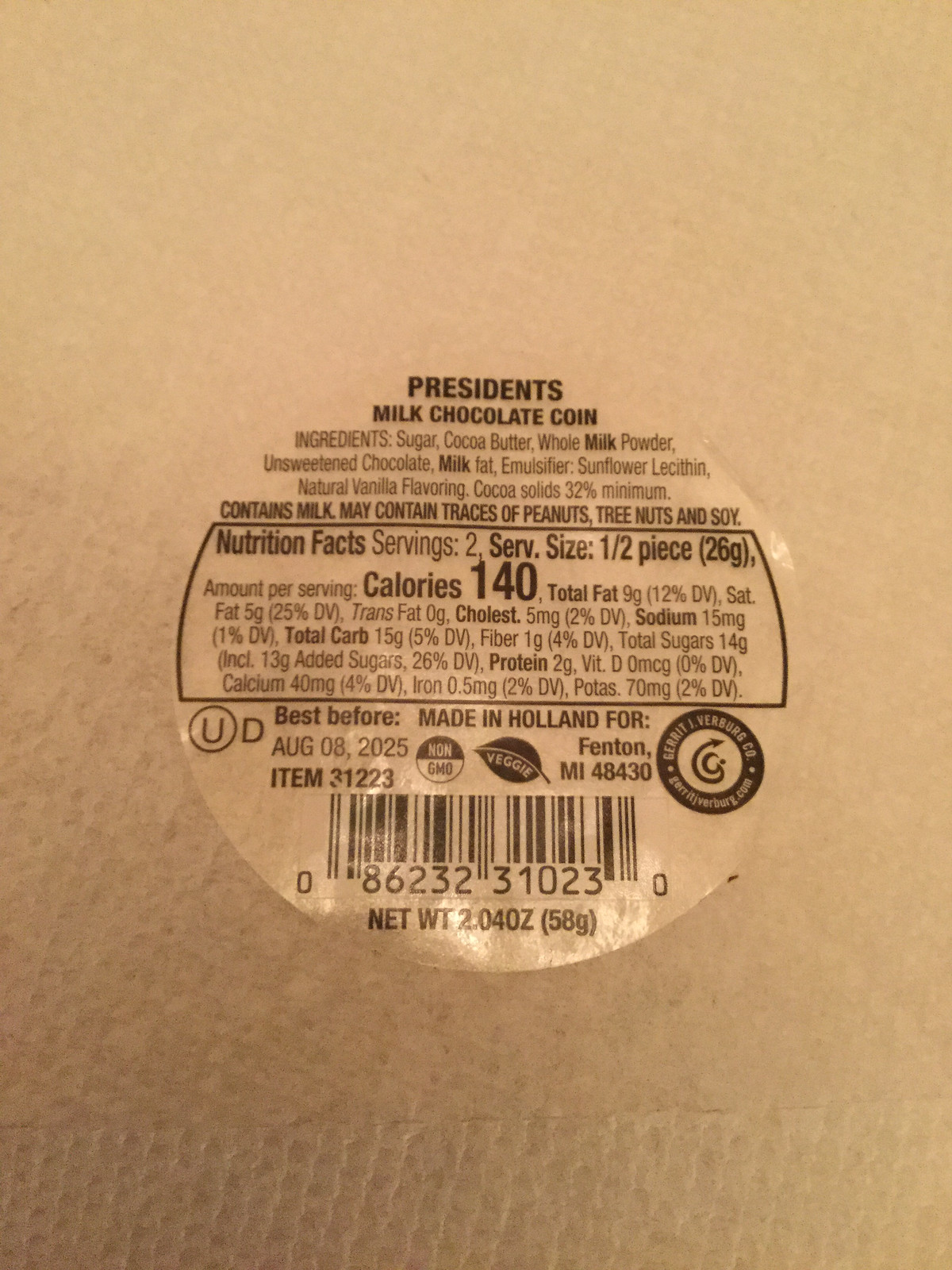This image features a detailed sticker label placed on a brown cardboard box. The sticker is clear with black text and prominently displays "President's Milk Chocolate Coin" in bold at the top. Below this, the label lists the ingredients: sugar, cocoa butter, whole milk powder, unsweetened chocolate, milk, sunflower lecithin, natural vanilla flavor, and cocoa solids with a minimum of 32%. It also notes that the product contains milk and may include traces of peanuts, tree nuts, and soy. A nutrition facts section provides detailed dietary information, indicating, for instance, that a half-piece portion contains 140 calories, totaling 280 calories for the entire coin. Additionally, the label includes a "best before" date of August 8, 2025, and features a barcode at the bottom. The background of the image transitions from a light tan at the top to a darker beige at the bottom, providing contrast to the sticker label.